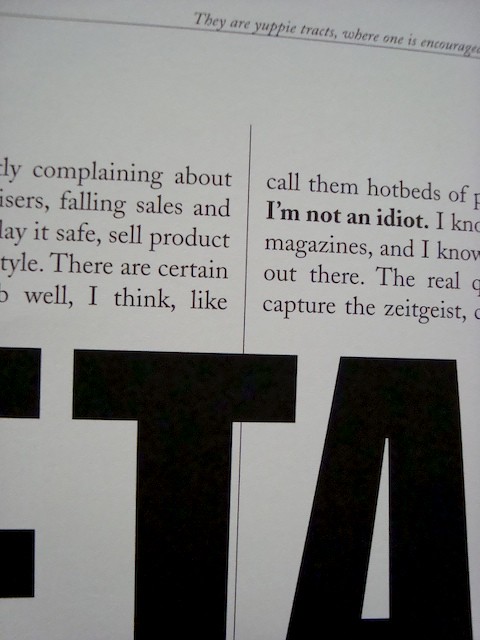The image appears to be a screenshot of a magazine article or a Kindle book page. The document is predominantly white with text broken into two columns and features a thin black dividing line near the top. Above this line, partial text reads "they are yuppie tracks where one is encouraged," though it is cut off. Below this line, the fragmented article includes phrases like "complaining about falling sales," "play it safe product," and "capture the zeitgeist." A highlighted section prominently states, "I am not an idiot." A large title appears in the middle, with "ETA" being the only discernible letters. The content seems to discuss topics related to business or sales, but the incomplete sentences make it difficult to ascertain the full context. There are no accompanying images.